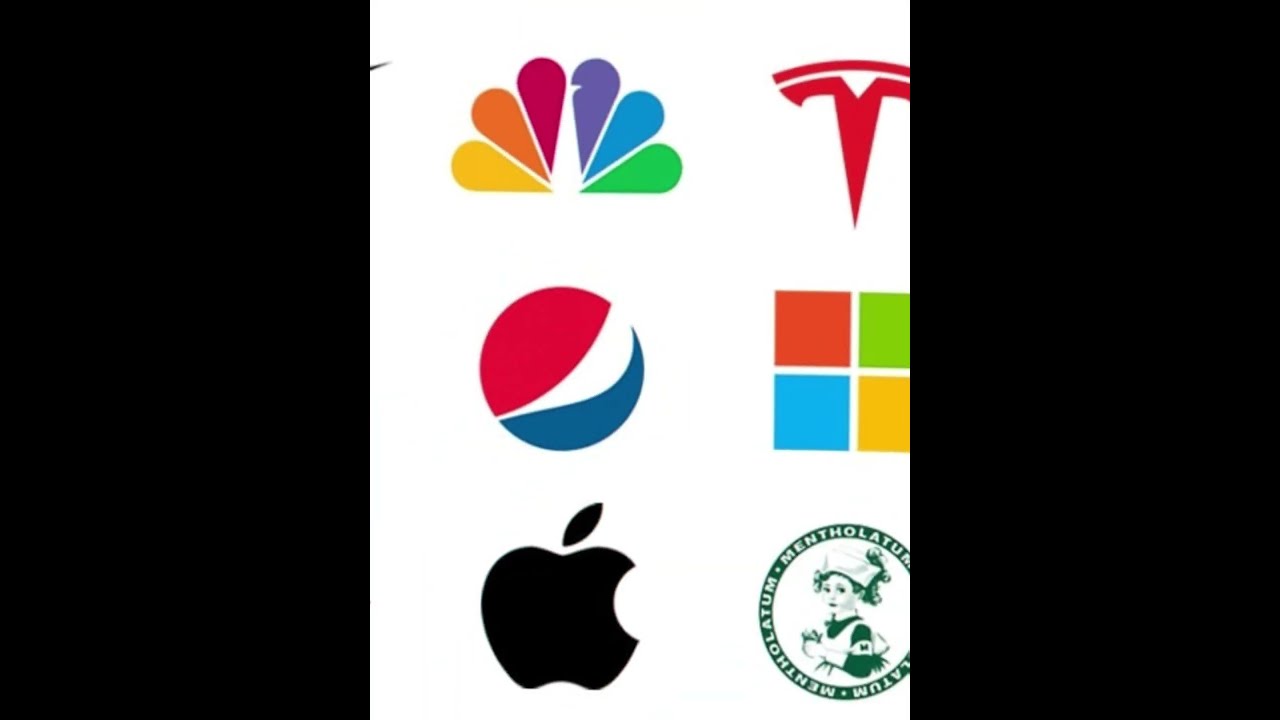This image is a detailed collage of various corporate logos set against a pristine white background, framed by a solid black border on both the left and right sides. In the top left corner, the NBC logo showcases its iconic peacock, composed of vibrant teardrop shapes in yellow, orange, magenta, purple, turquoise, and telly green, representing the peacock's fanned tail. To its immediate right, the Tesla logo features a sharp, arrow-like capital 'T' with a gracefully curved top.

In the middle row, starting from the left, the Pepsi logo appears as a divided circle with a red top half, a white wavy strip in the center, and a navy blue bottom half. Adjacent to it on the right is the Microsoft logo, a grid of four squares in distinct colors: a red square at the top left, a green square next to it, a blue square beneath the red, and a yellow square next to the blue.

At the bottom left, the Apple logo is a sleek silhouette of an apple with a characteristic bite taken out, including a small black stem. In the bottom right corner, there's a less familiar logo: a circular emblem featuring a young girl dressed as a nurse with the text 'Mentholatum' encircling it, primarily in green.

The image contains no text outside the logos themselves, and the color palette spans black, white, yellow, orange, magenta, purple, blue, green, red, and golden hues, providing a rich visual diversity. Overall, it presents a well-organized and vivid representation of globally recognized brands.